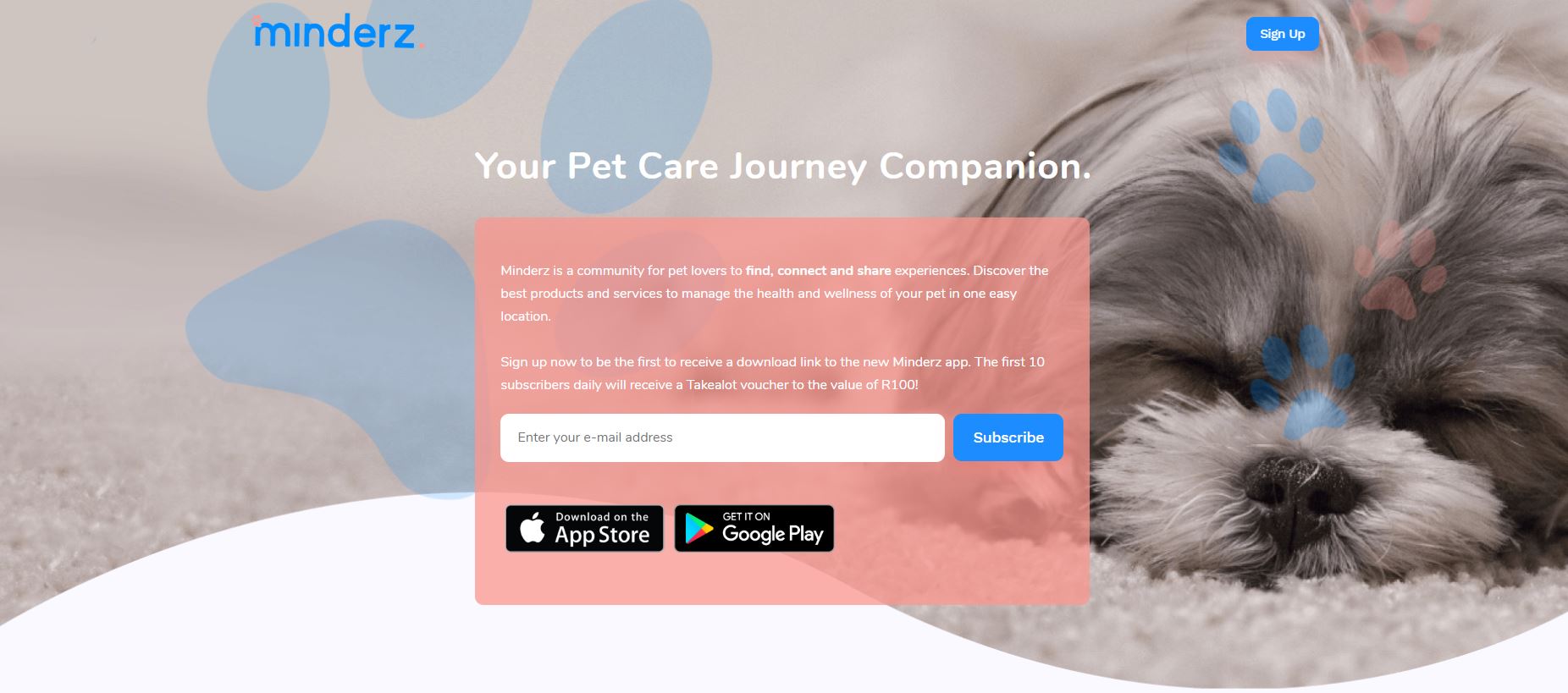The image showcases a website entry for a pet care platform called "Minders." The focal point of the visual is an adorable dog, peacefully napping on an immaculate white carpet. The dog's face is in close-up, with its eyes closed and its chin resting on the plush carpet. The dog's nose is black, and its fur features a charming palette of white and light charcoal gray, particularly around its jaw and eyes. Strands of white and gray fur blend seamlessly as the body moves out of the camera's frame.

Behind this endearing image, there is a large blue paw print, reinforcing the pet-centric theme of the website. Below the paw print, the text reads, "Your Pet Care Journey Companion." Further down, a prominent peach-colored section describes the purpose of Minders: "Minders is a community for pet lovers to find, connect, and share experiences. Discover the best products and services to manage the health and wellness of your pet in one easy location." Users are encouraged to sign up via a button at the top of the page, where they can enter their email address. Additionally, the website offers app downloads available on the App Store and Google Play, promising an integrated solution to help pet owners care for their furry friends.